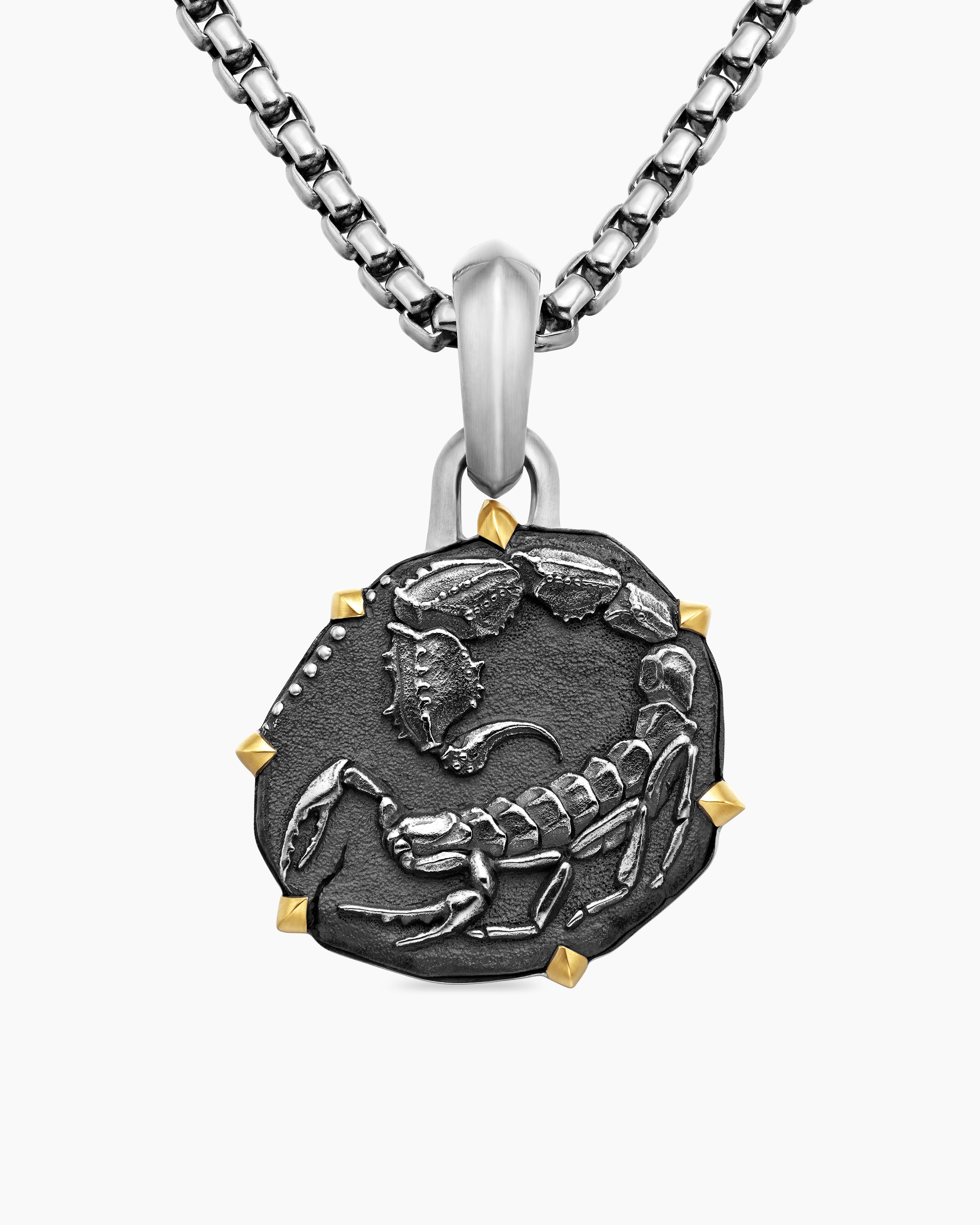The color photograph, set against a white background, showcases a detailed scorpion necklace. The necklace features a silver chain with rectangular interconnected links, coming from both sides at the top. Attached to the chain is a round, albeit slightly irregular, darker silver pendant. This pendant bears a raised depiction of a scorpion, whose lighter silver body is intricately designed with its end barb in the center, curving upwards, then to the right, and finally downwards to face left, displaying prominent pincers. The pendant is further adorned with seven gold, seed-like dots around its outer edge. Between some of these gold dots, smaller silver dots add extra detail, enhancing the pendant's elaborate design.